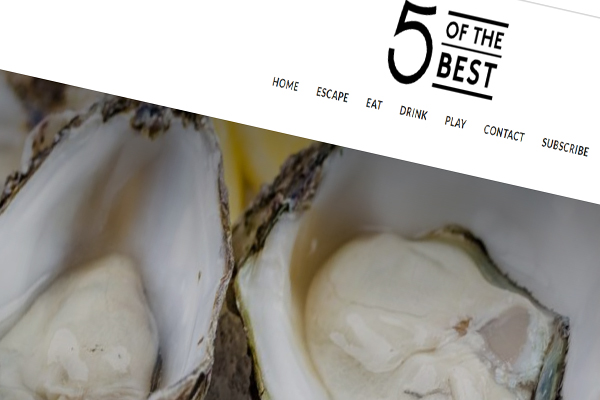This slightly skewed image, likely from a cooking website or restaurant, features a dynamic and engaging layout. In the top right corner, bold black text declares "Five of the Best," with "Five" standing out prominently in large font. The words are separated by a series of horizontal lines: a thick black line at the top, a thinner black line in the middle accompanying "of the," and another thick black line underlining "best." Below this striking heading, seven navigation tabs—Home, Escape, Eat, Drink, Play, Contact, and Subscribe—are neatly aligned in black text on a white background.

Dominating the visual is a close-up photograph of freshly shucked oysters. Their pearly white inner shells contrast vividly with their rugged, brown, grey, and black exteriors. The soft, delicate flesh of two oysters is particularly prominent, highlighting their fresh, tender appeal. This exquisite image is enticingly detailed, capturing the textural interplay of the oysters and inviting viewers to savor their natural beauty.